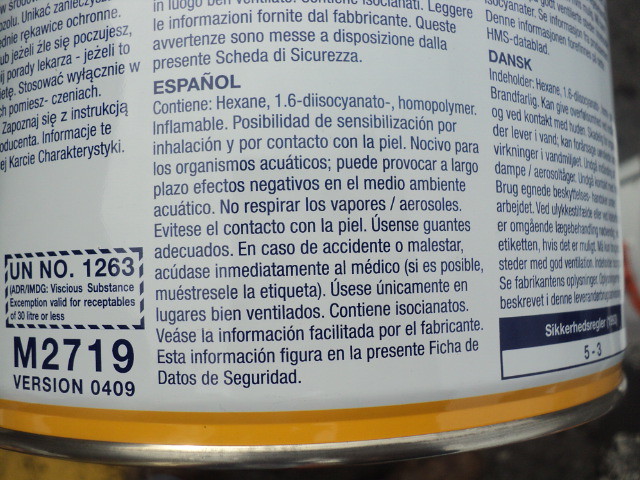A photograph captures the back of a cylindrical product can. The image reveals a bottom section featuring a prominent silver band. Directly above this, there is a yellowish band, followed by a white section adorned with navy blue text. The text includes alphanumeric codes "VERSION 0409" and "M2719" towards the bottom. Writing in Spanish is also visible on the back of the can, though the specific contents remain unclear. Additionally, the side of the can displays the numbers "5-3." The can appears to be of a large size, and a slight white reflection can be seen near its base. The absence of a front label or any identifying features makes it challenging to ascertain the product's exact identity.